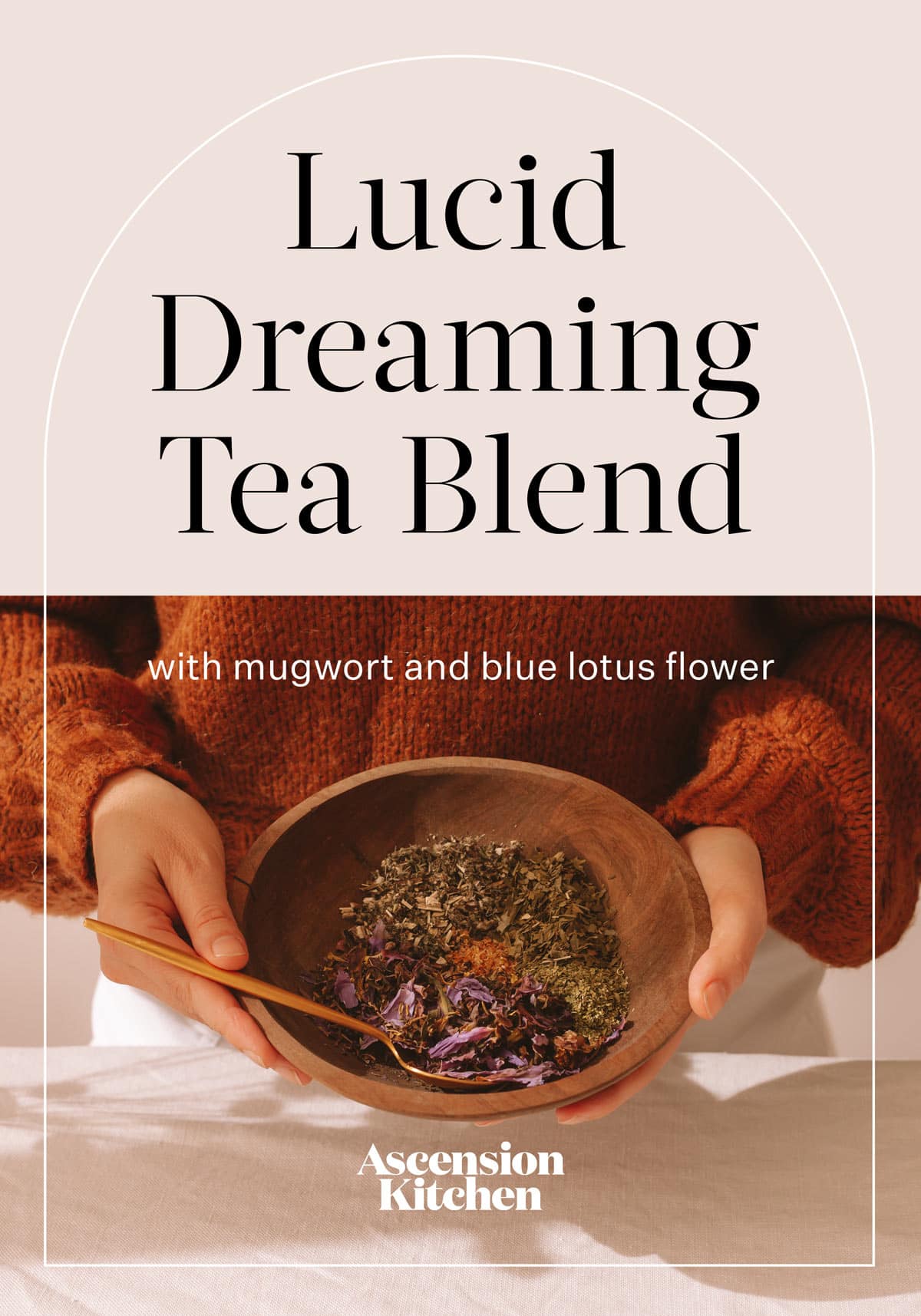The image appears to be a highly detailed promotional cover, likely for a product such as a tea blend. It features a light grey-white background with prominent large black text at the top that reads "Lucid Dreaming Tea Blend." The bottom section showcases a person wearing a burnt orange sweater, visible from the belly button to the top of the thighs, holding a wooden bowl with both hands. Inside the bowl are various herbs, including green, purple, and orange powders, signifying mugwort and blue lotus flower among other ingredients. There is also a wooden-handled spoon in the bowl, as if the person is about to mix the tea blend. The setup is placed on a white, possibly white marble, kitchen counter. At the very bottom of the image, the text reads "Ascension Kitchen," indicating the brand associated with the product.